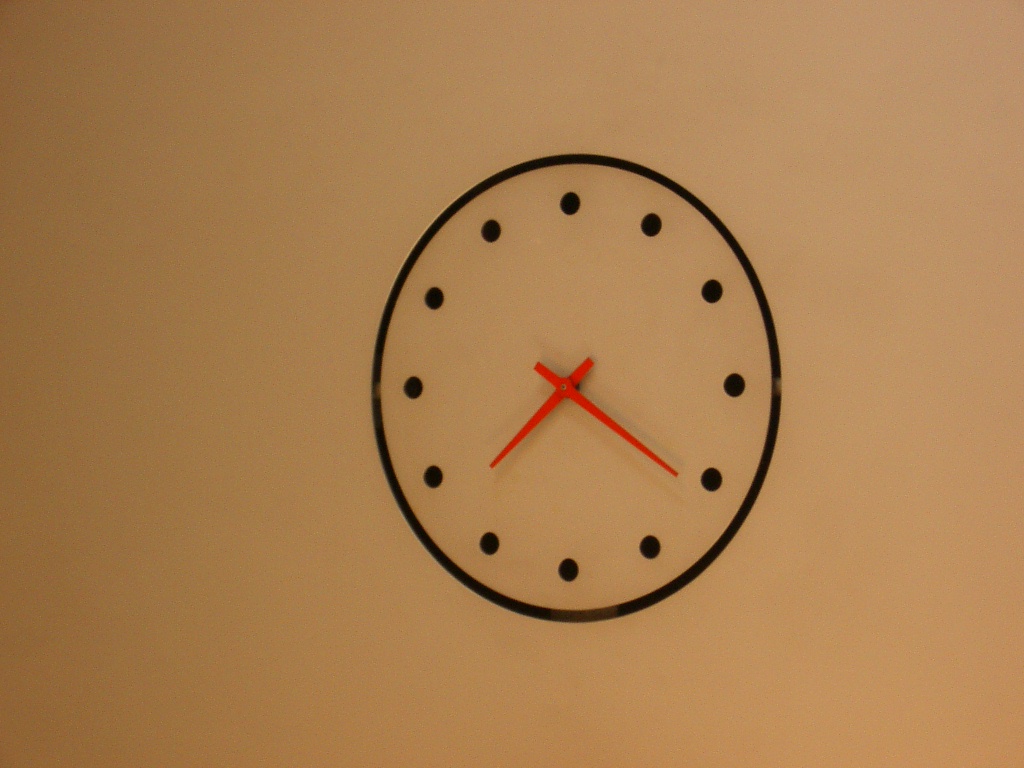This detailed image depicts a minimalist clock set against a beige wall. The clock features a black see-through outer circle with twelve black dots indicating the hours, lacking any numerical labels. The hour and minute hands, colored in a deep lipstick red, point to approximately 7:21. While the clock appears to be a standard 12-hour analog design, there are no visible mechanisms, suggesting it could be a drawing rather than a functioning timepiece. This flat representation on the wall might also include hands made from glued or taped materials, possibly used for educational purposes. The entire setup gives the impression of a simple, artistic, or instructional clock.